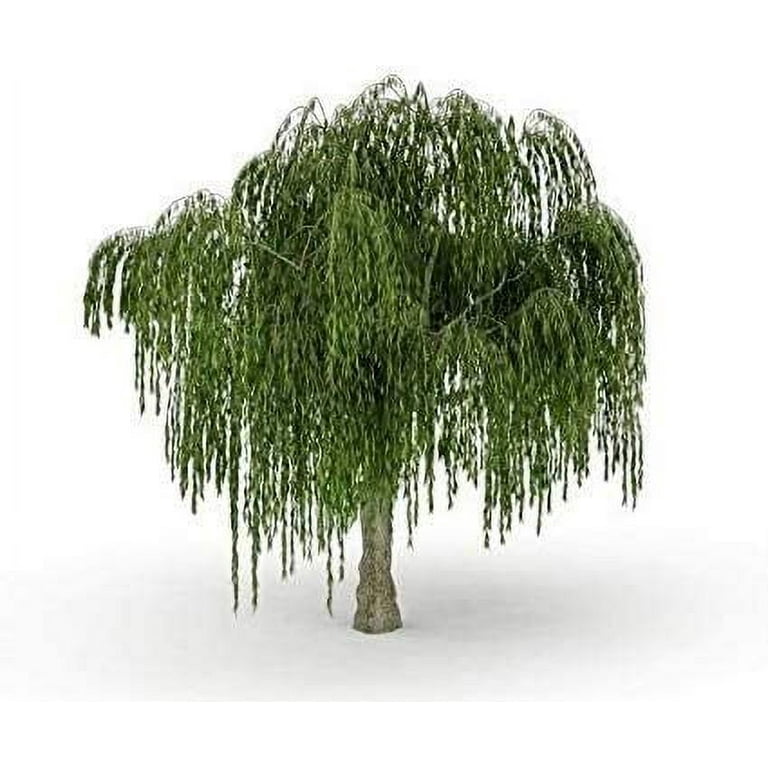This image features a tall, decorative tree with a cascade of long, drooping branches and leaves, resembling a willow tree. The tree appears digitally created or heavily edited, placed against a blank white background, suggesting it has been photoshopped out of its original setting. The photo is in portrait orientation and of somewhat low quality, with visible pixelation. The leaves, colored a pine tree green, hang down almost to the bottom, creating an umbrella-like canopy. The tree lacks visible roots and ends abruptly at the ground. It seems a bit neglected and could benefit from pruning to enhance its health and appearance.